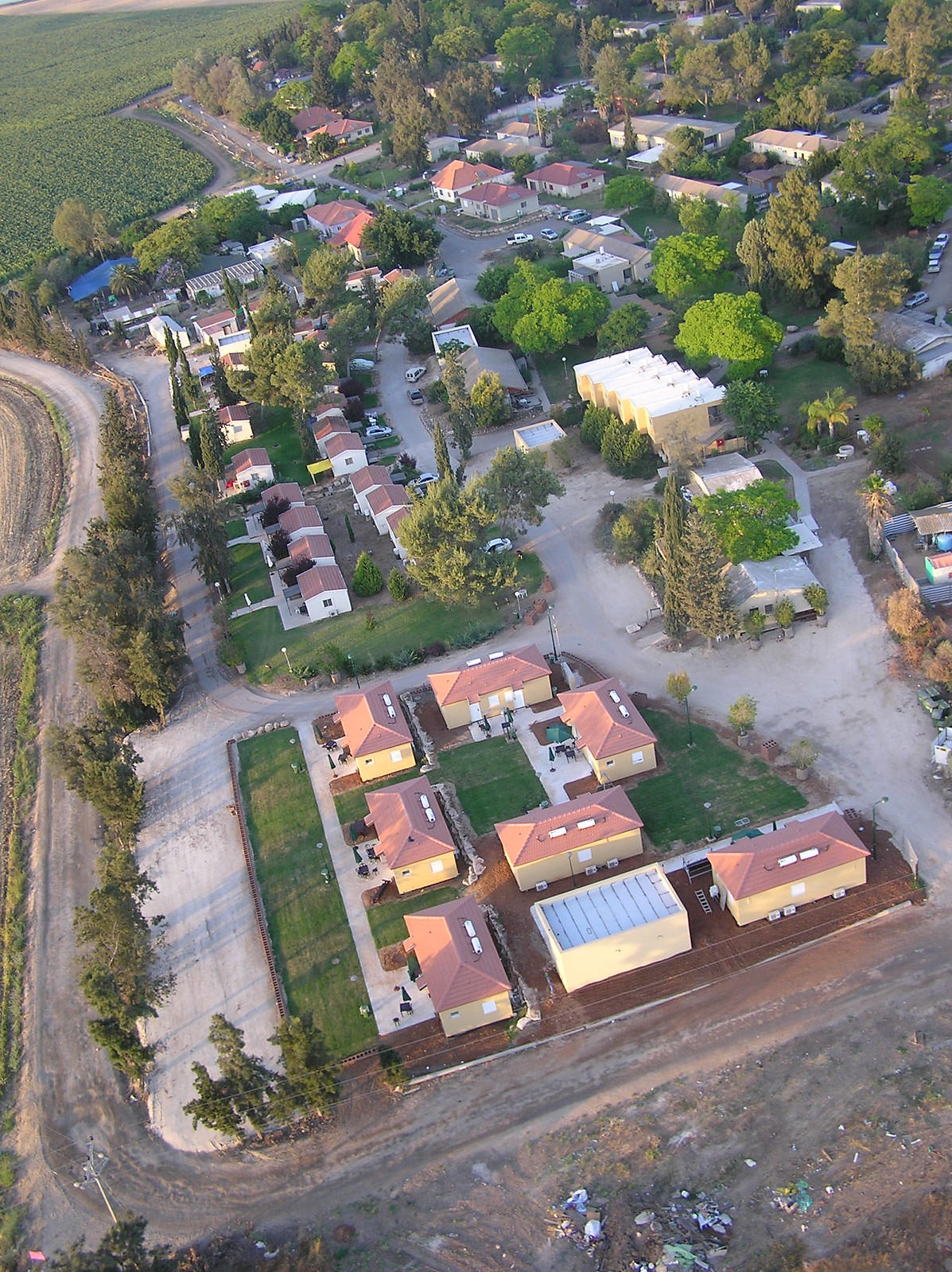This detailed aerial photograph captures a small suburban neighborhood surrounded by both farmland and undeveloped land. In the top left corner, neat rows of green crops are visible, indicative of rural farm fields. Dominating the middle and right sections of the image, a series of identical rectangular houses with reddish-brown or terracotta roofs, well-maintained green lawns, and scattered trees can be observed. There is a distinct pie-shaped section with uniform houses in the center. Along the bottom and left side of the photograph, a dirt road is winding its way around the neighborhood, creating a perimeter and transitioning into some paved sections. In the bottom right, an area of exposed dirt can be seen, with a small garbage dump nearby. Additionally, one of the houses features a swimming pool, adding a unique detail to the uniformity of the neighborhood.